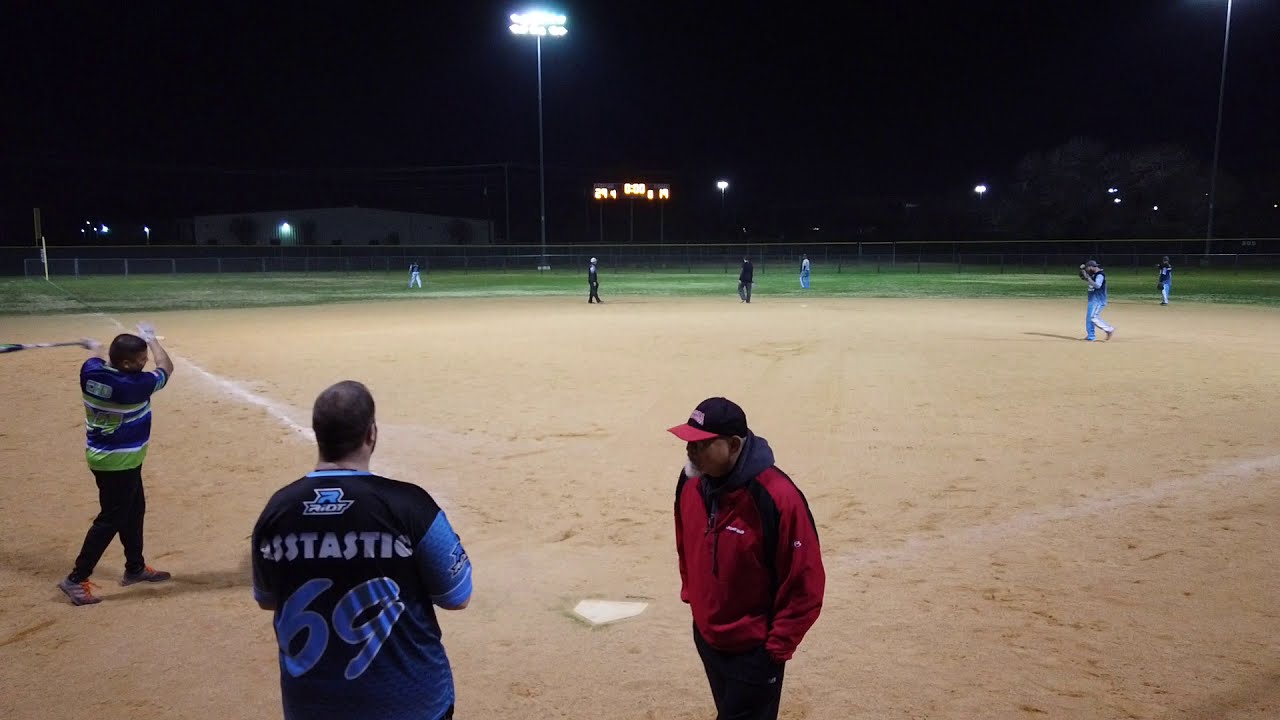This horizontal rectangular photograph captures a nighttime baseball game viewed from behind home plate, likely taken by someone in the bleachers given the elevated angle slightly above the players' heads. The field is well-lit by surrounding lights, highlighting a green grassy outfield and a beige, dusted infield with white bases. 

In the foreground, a man holding a bat on the left is dressed in a blue, white, and green jersey paired with black pants, suggesting it's his turn to bat next. Near the center of the photo, another individual clad in a red hoodie, with a black baseball cap featuring an unreadable red and white logo, appears to be a coach. This man, who seems to be over 35 years old and obese, is talking to a player on his team who has "Ass-tastic 69" and "Riot" along with an R logo on his jersey. The informal attire and mixed team jerseys hint at this being a recreational or company-organized game. In the background, players are scattered across the field, ready for the next play, all set against the black night sky.